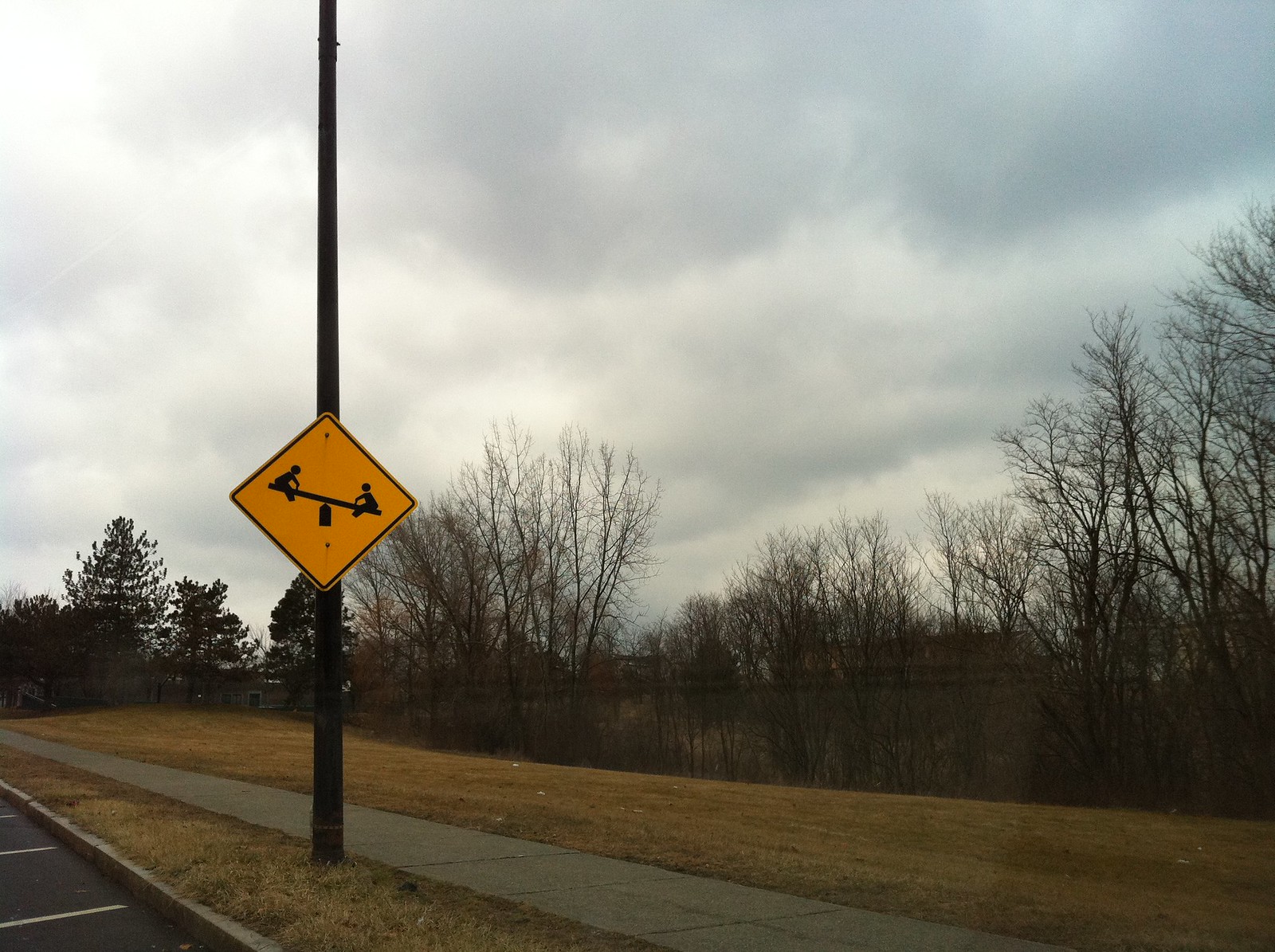A low-hanging, diamond-shaped street sign mounted on a dark pole stands prominently in a parking lot, clearly visible due to its unusual height. The yellow sign features an illustration of two children on a seesaw, leaning slightly to the right. Surrounding the sign are standard white parking space dividers that lead directly to a nearby curb and sidewalk. The image appears to be taken from inside a car, with a faint shadow of the windshield and bare trees in the background suggesting a fall or winter scene. The overhead sky is heavily clouded and gray, contrasting with the towering evergreens nearby, adding to the dreary ambiance of the setting.